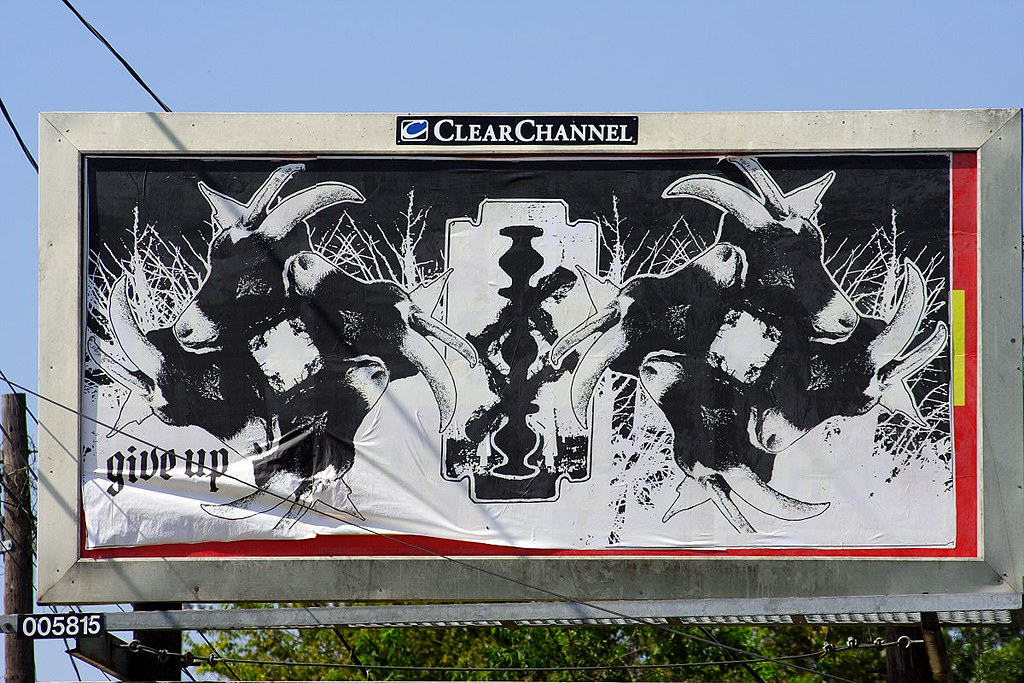This image captures a creatively altered billboard. The primary feature of the billboard is an illustration of several goats' heads, arranged in a circular pattern and repeated twice. Each circular icon is composed of four goats' heads, artistically tilted to form the shape of a circle. Across this graphic, the bold words "GIVE UP" are prominently displayed. It appears that this particular sign was placed over an original red billboard, which is partially visible beneath the newer overlay. This suggests that the current sign might be an act of subversive art rather than sanctioned advertising. The billboard is owned by Clear Channel, as indicated by the company's name on the border. In the background, trees and a clear sky provide a natural frame to the scene.